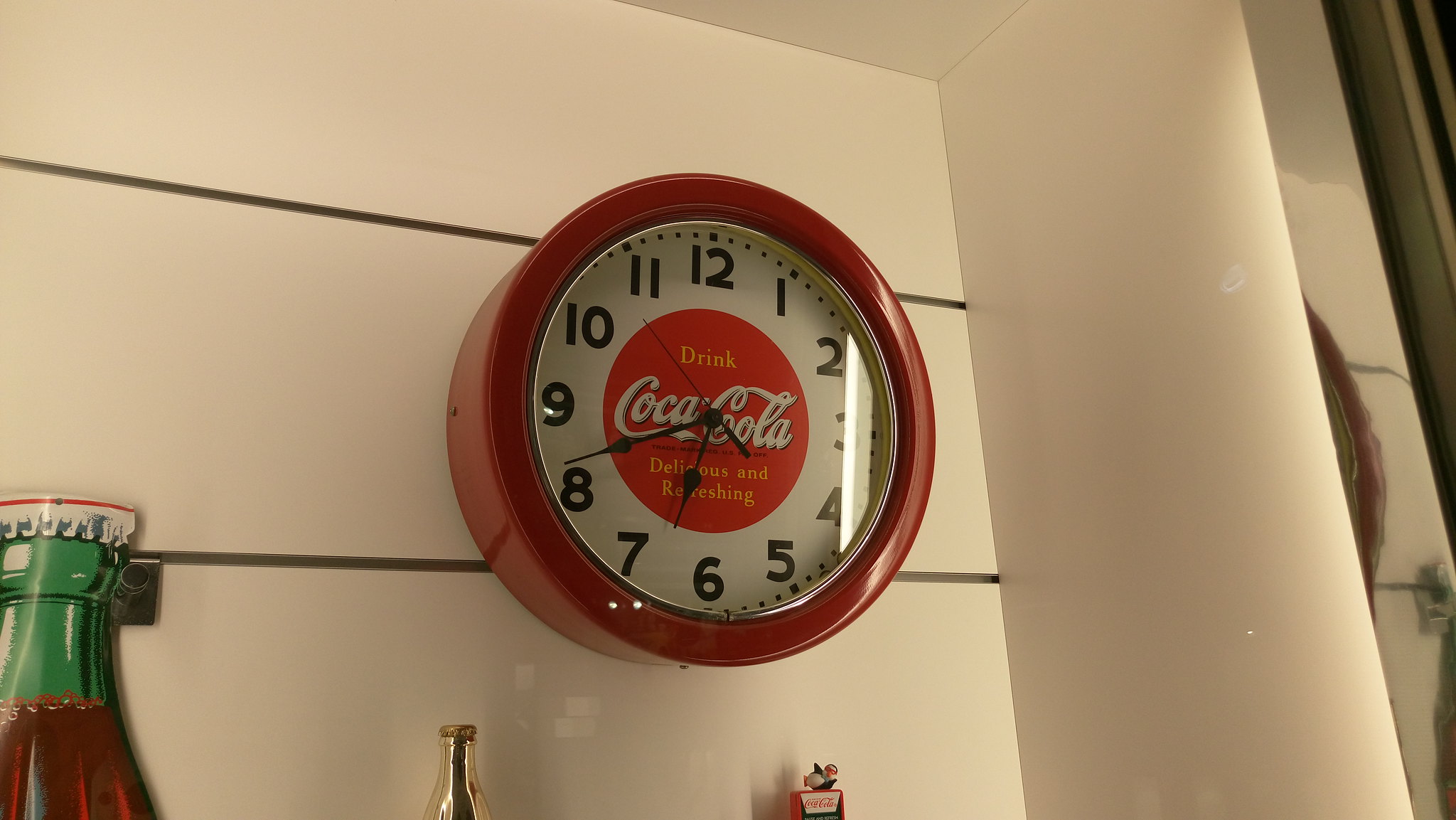This is an image featuring a retro-style, circular Coca-Cola wall clock. The clock is prominently displayed on a beige wall with a beige column in front. The clock has a thick red edge framing a predominantly white and red face. Black numbers encircle the clock, with dotted minute markers, and black hands indicating the time at approximately 6:42. 

At the center of the clock's face is a striking red circle with the iconic Coca-Cola logo. Within this circle, "Drink" is written in orange, followed by "Coca-Cola" in bold white letters, and below that, "Delicious and Refreshing" also in orange. 

On the lower segment of the image, additional Coca-Cola memorabilia are visible. The bottom-left corner features an artistic representation of a Coca-Cola bottle cap, a green bottle neck, and a small portion of the bottle appearing brown. Just to the right of this, there is a silver-colored bottle, and a red object, possibly another piece of Coca-Cola themed decor. The clock is mounted on a white paneled wall, adding to the vintage aesthetic of the scene.